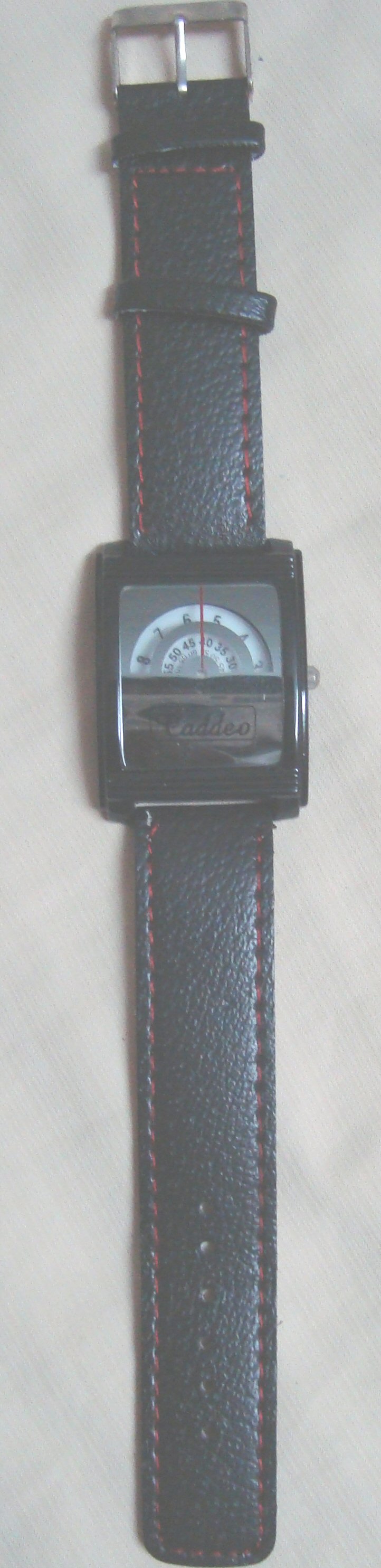The image depicts a sophisticated timepiece centered against a neutral grey background. The watch features an elegant black leather band, accompanied by a sleek silver metal fastener. The most striking aspect of the design is the semi-circular watch face, which deviates from traditional full-circle watch faces. The outer rim of the semi-circle is adorned with clearly visible white numerals. Within this, there is a smaller white circle, serving as the core of the dial, surrounded by a grey accent. A vivid red streak cuts through the middle, adding a bold touch of color. The watch is equipped with a small, refined silver winder for adjustments. The leather band has meticulously punched holes at the far end, ensuring a perfect fit when the buckle is fastened. Overall, the image captures a blend of modern design and classic detailing in a sophisticated and stylish watch.